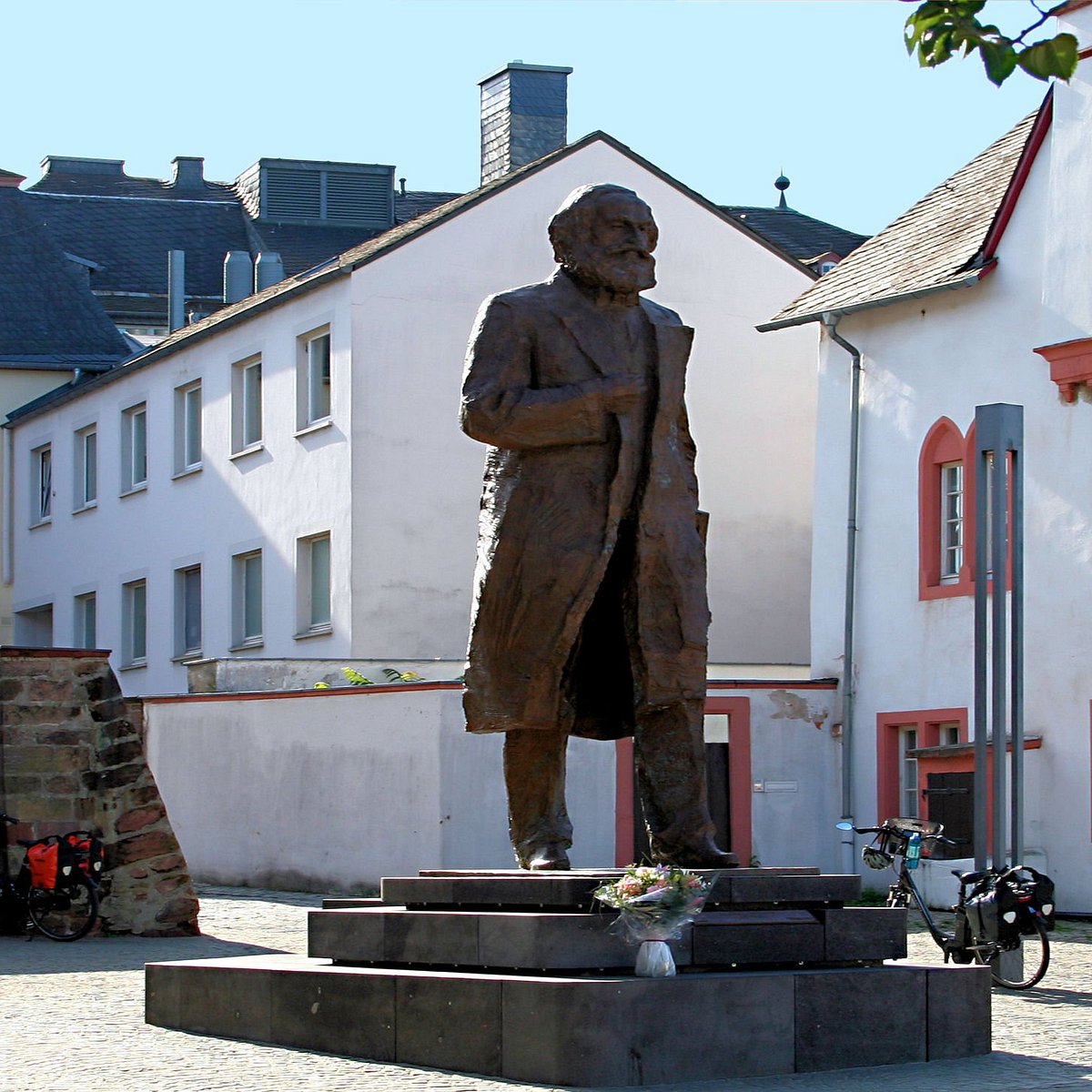The photograph captures a detailed and compelling scene centered around a bronze statue of an older, bearded man donning a trench coat, pants, and boots. The statue, which is brown in color, portrays the man with his hand on one of his lapels, possibly in a walking pose, and stands on a multi-stepped podium. A bouquet of flowers is carefully placed at the base of the podium. The background reveals a charming European town with predominantly white stucco buildings featuring reddish-pink accents around the windows and doorways, creating an old-world ambiance. There are several bicycles in the vicinity, including one with a helmet hanging from the handlebar and another equipped with red and black saddlebags leaning against a stone ledge wall to the left. No people are visible in the photograph, emphasizing the tranquility and historic feel of the setting.